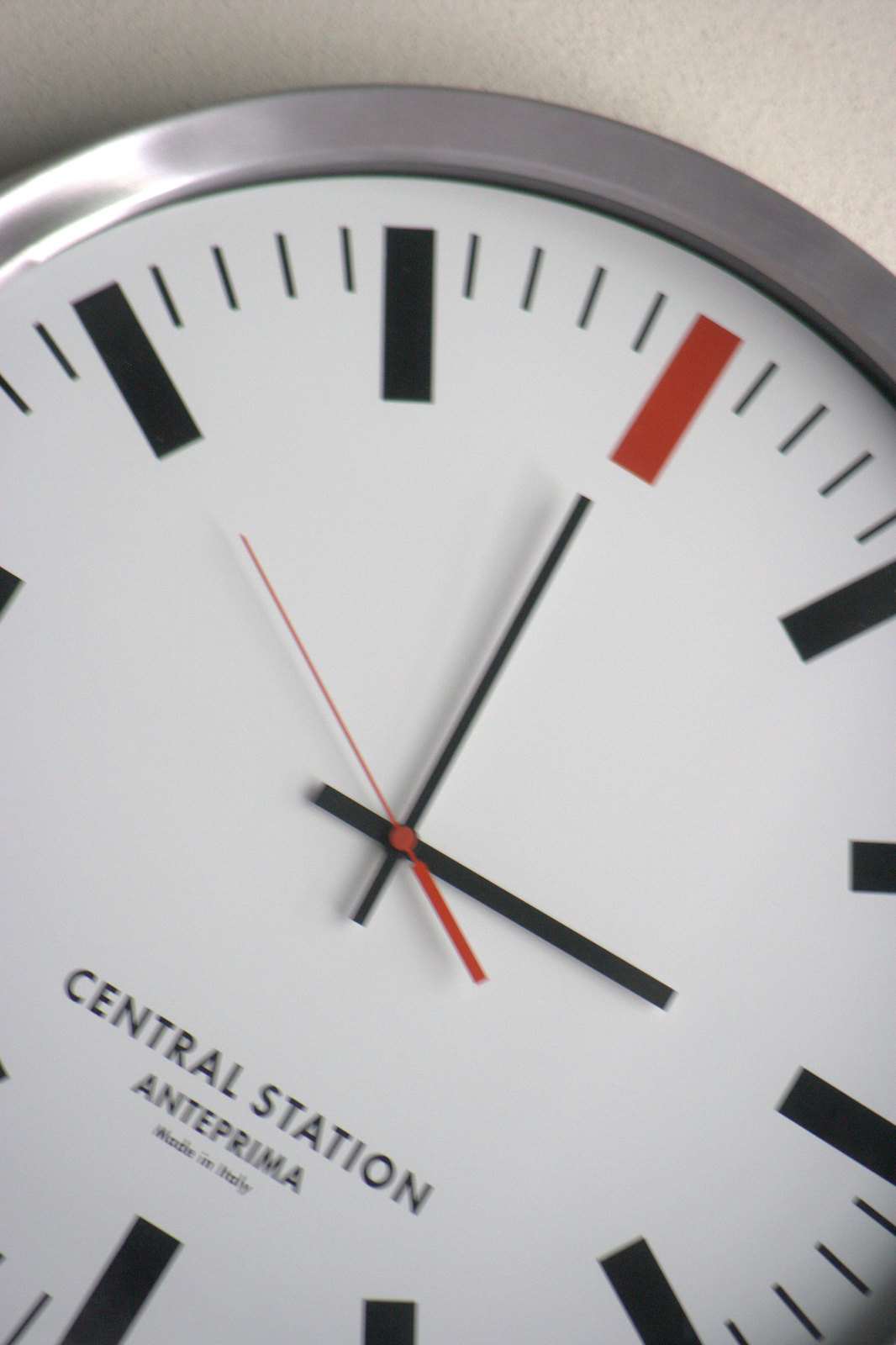This close-up photograph features an analog clock mounted on a textured white surface. The clock, with its silver border, has a clean white face devoid of numbers, instead marked by thick vertical black lines for the hours and thinner vertical black lines for the minutes. The 12 o'clock position is uniquely highlighted with a prominent red rectangle. The clock hands are black, with the minute hand pointing at 2 and the hour hand pointing at 3, indicating a time of 3:10. In the center of the clock face, the words "Central Station" and "A-N-T-E-P-R-I-M-A" are displayed in black, with "Made in Italy" written beneath them. This elegant design is accentuated by the clock's minimalist aesthetic and precise detailing, making it a striking yet straightforward depiction of time.